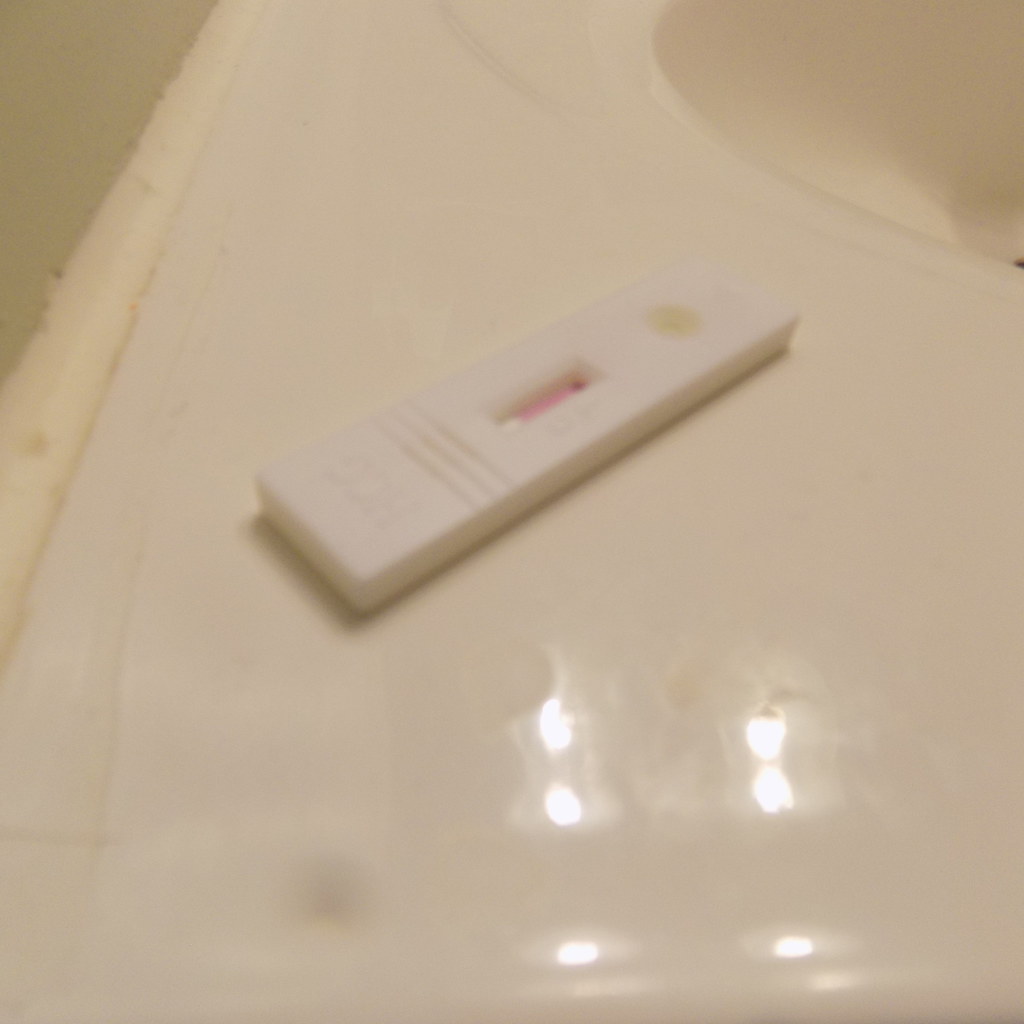The image depicts a small rectangular pregnancy test placed on a white bathroom sink. The sink stretches across the bottom of the frame and extends upward about two-thirds of the way into the image. Positioned diagonally, the pregnancy test points from the bottom left corner toward the upper right corner.

In the top left corner, a small triangular section shows the wall or floor in a brownish-white color. Additionally, a thin, dingy white border is visible running from the top left and going midway down the left side, separating the wall from the rest of the sink.

In the upper right section, the sink's hollow, pristine white basin is clearly visible, extending about three inches from both the top and the right edges. There are no objects within this part of the sink.

Positioned at the bottom left of the image, the pregnancy test's bottom end angles diagonally toward the upper right corner. The test's casing has three horizontal indentations about an inch from its bottom end. The long rectangular test strip features a window near the middle where the result is displayed, which is colored pink. There is a small brown spot at the tip of the test, likely where the urine sample was applied.